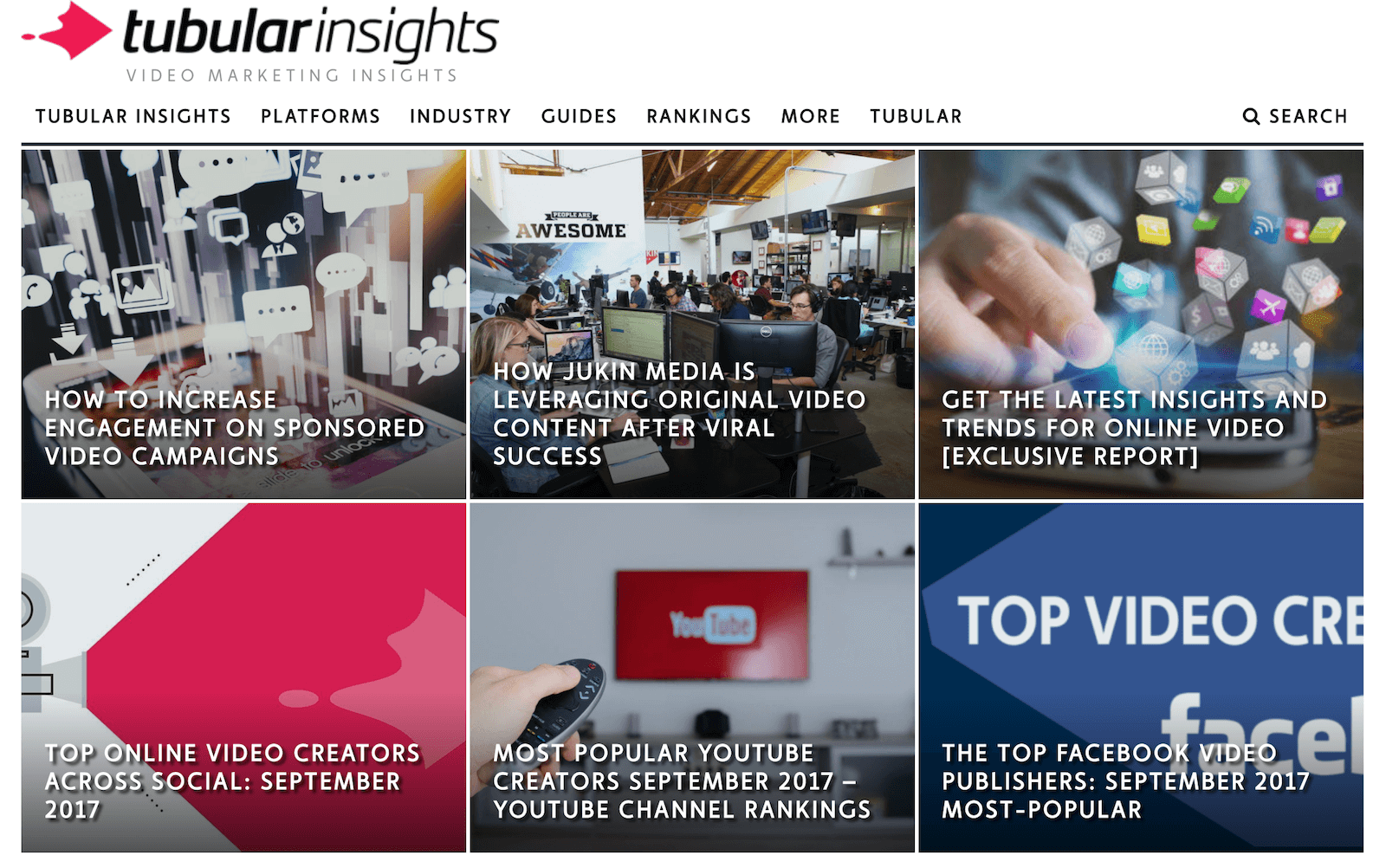This image, sourced from the website Tubular Insights, features a comprehensive layout of video marketing insights. The title "Video Marketing Insights" is prominently displayed, with "Tubular" written in black and "Insights" in gray. An emblem resembling a right-turned kite, depicted in red, provides a visual accent to the display.

At the top of the image, menu categories including "Categories," "Tubular Insights," "Platforms," "Industry," "Guides," "Rankings," and "More" are listed, along with another "Tubular" link. On the right-hand side, there is a search bar with the label "Search" and an accompanying magnifying glass icon.

The central section of the image features six distinct sections:

1. The first section is titled "How to Increase Engagement on Sponsored Video Campaigns" and is accompanied by an image of various video icons floating in the air.

2. The second section, "How Jukin Media is Leveraging Original Video Content After Viral Success," depicts a spacious room filled with numerous individuals working on computers.

3. The third section, "Get the Latest Insights and Trends for Online Video Exclusive Report," features an image of a person’s hand appearing to juggle multiple colored dice-like icons in vibrant hues such as purple, green, blue, pink, and yellow.

4. The fourth section is titled "Top Online Video Creators Across Social, September 2017," without an accompanying image description.

5. The fifth section reads "Most Popular YouTube Creators, September 2017 – YouTube Channel Rankings."

6. The sixth section, though partially cut off, seems to describe "Top Video Creators" on Facebook, with a focus on the most popular Facebook video publishers from September 2017.

This layout serves as an engaging overview of current trends, guides, and rankings in the video marketing industry.